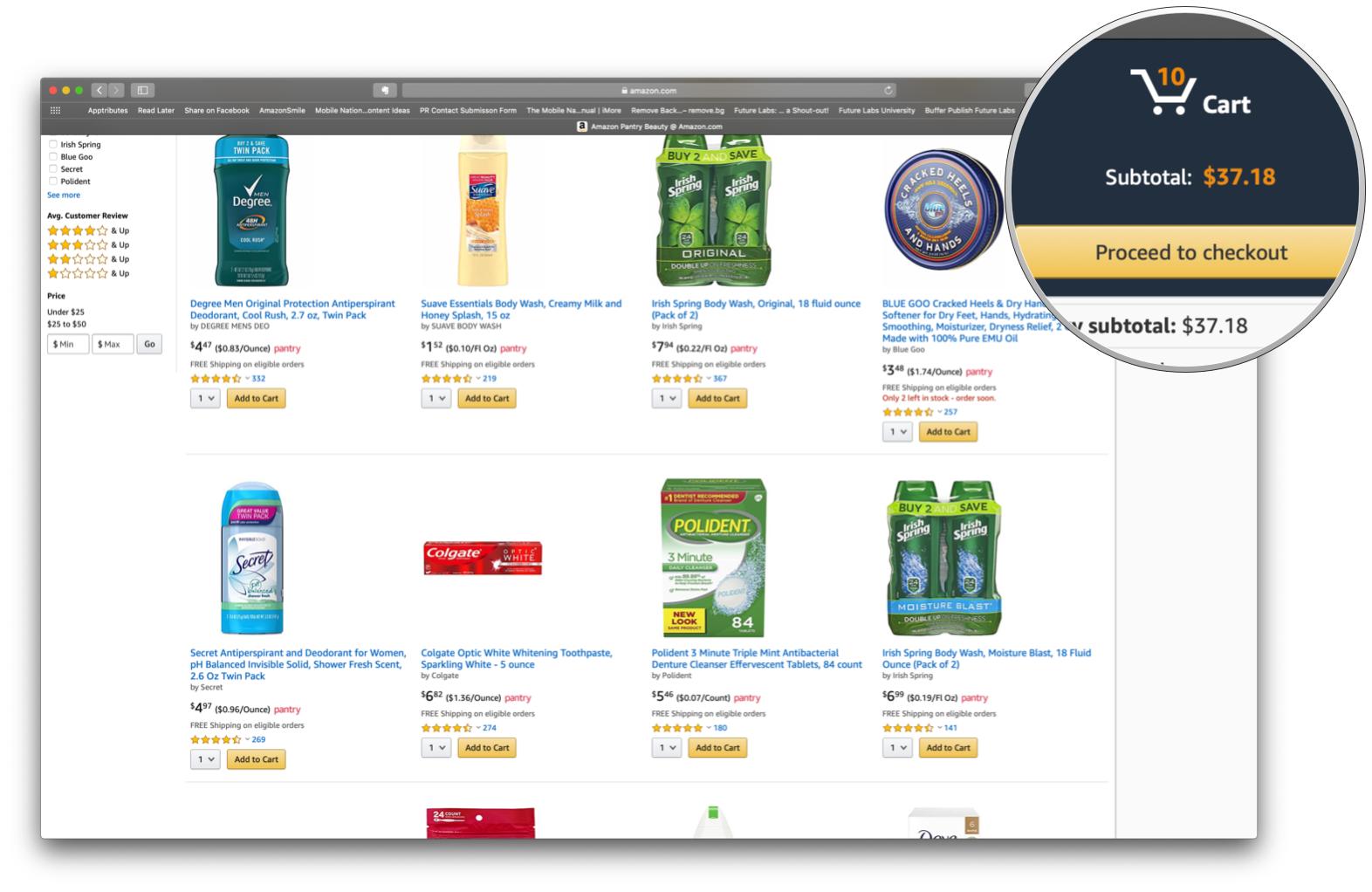This detailed descriptive caption describes a screenshot of the Amazon.com website displayed in a web browser with a highlighted section:

The Amazon.com webpage is open in a web browser, characterized by its predominantly white background and a dark grey header. At the top of the screen, a light grey search bar displays "Amazon.com" in white text, accompanied by a white lock icon to the left of the text, signaling a secure connection.

Below the header, products are presented in a grid layout, each with an accompanying image, product name in blue text, price, reviews, and action buttons. Each product entry features a yellow 'Add to Cart' button in the bottom right corner and a quantity selector with a default value of '1' and a grey arrow pointing downwards for adjustments.

The products featured in the top row, from left to right, are:
1. Degree Men Original Protection Antiperspirant Deodorant, Cool Rush 2.7oz Twin Pack
2. Suave Essentials Body Wash, Creamy Milk and Honey Splash, 15oz
3. Irish Spring Body Wash, Original, 18 fluid ounces, Pack of Two
4. Blue Goo Cracked Heels & Dry Hands Softener for Dry Feet & Hands, Hydrating, Smoothing Moisturizer for Dryness Relief, 2oz, made with 100% pure emu oil (text is cut off).

The second row of products includes:
1. Secret Antiperspirant Deodorant for Women, pH Balanced, Invisible Solid, Shower Fresh Scent, 2.6oz Twin Pack
2. Colgate Optic Whitening Toothpaste, Sparkling White, 5oz
3. Poligrip 3-Minute Triple Mint Antibacterial Denture Cleanser Effervescent Tablets, 84 count
4. Irish Spring Body Wash, Moisture Blast, 18 fluid ounces, Pack of Two.

A highlighted section of the screenshot is displayed in a magnified view with a silver outline. This close-up highlights a white cart icon with an adjacent "Cart" label and an orange "10" indicating the number of items. Beneath this, "Subtotal:" is shown in white text, followed by the subtotal amount in orange, "$37.18." Directly below this, a yellow button with black text reading "Proceed to Checkout" is visible.